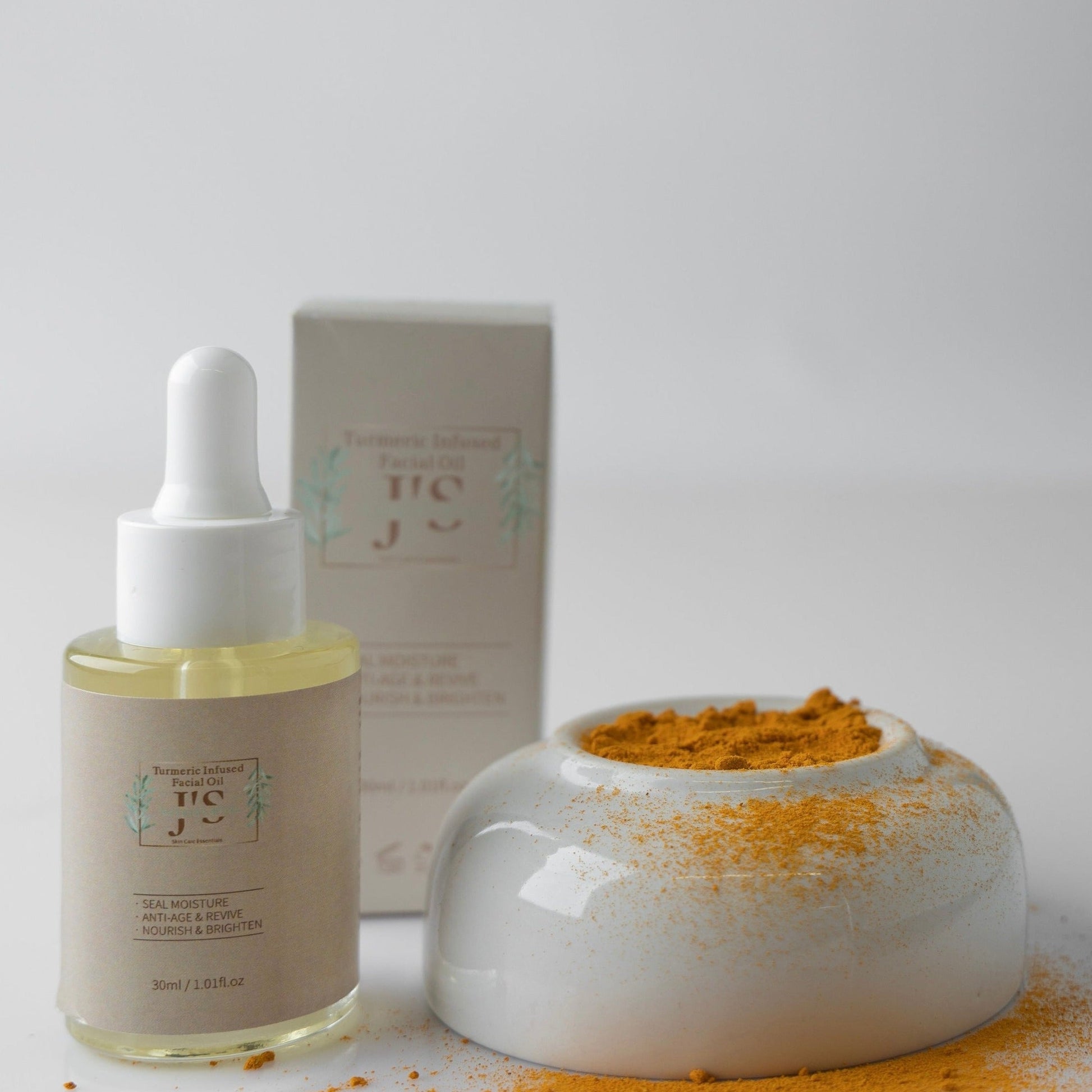The image is an advertisement for a skincare product featuring a Turmeric-Infused Facial Oil. Set against a white background and surface, the composition includes three items: a clear glass bottle with a white squeezable dropper, a matching box, and a white dish filled with vibrant orange powder. The bottle, labeled with a tan square adorned with green leaves, prominently displays "Turmeric-Infused Facial Oil, J's" along with benefits such as "Seal Moisture," "Anti-Age and Revive," "Nourish and Brighten," and the quantity "30 mL / 1.01 fl oz." Overlapping with the dish, some of the turmeric powder has spilled onto the surface, adding a tactile element to the visual. The accompanying box shares the same label details but appears slightly blurred in the background, emphasizing the bottle and dish in the foreground.